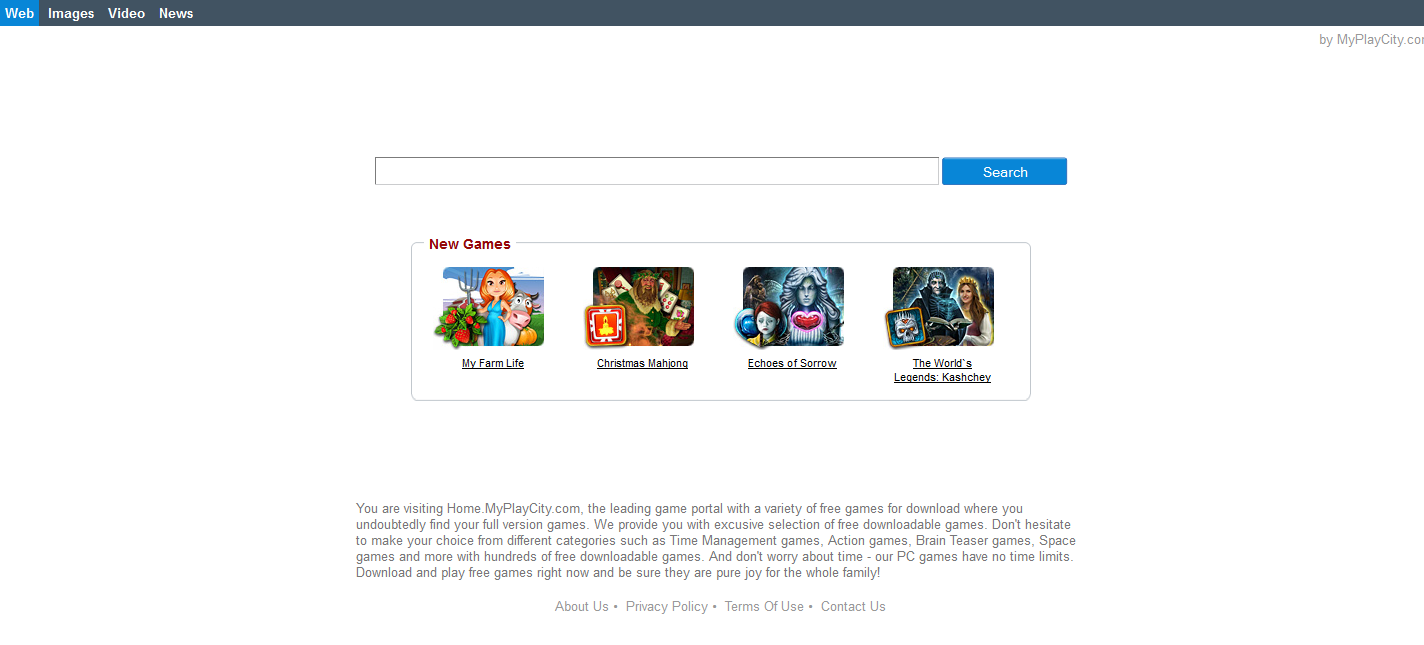The image displays a desktop screenshot of a minimally designed website. The toolbar at the top is a dark grayish-blue, featuring small print options: "Web," "Images," "Video," and "News," with "Web" currently selected. The webpage background is a clean white, highlighted by a long search bar at the top and a prominent blue search button. Below the search bar, there is a rectangular section showcasing four game thumbnails under the title "New Games." These games are:

1. **My Farm Life** - Illustrated with a woman in a dress, accompanied by a cow, plants, and a pitchfork.
2. **Christmas Mahjong** - A festive mahjong game.
3. **Echoes of Sorrow** - A game likely centering on a sorrowful or eerie theme.
4. **The World's Legends: Kashchey** - Depicting elements of legend or folklore.

The website being visited is "home.myplaycity.com," identified as a leading game portal offering a variety of free downloadable games. The site boasts an exclusive selection, encouraging users to explore different categories such as time management games, brain teasers, and space games, among others. It emphasizes that all PC games available come with no time limits, making them perfect entertainment for the entire family. The website invites users to download and enjoy pure, unrestricted gaming joy.